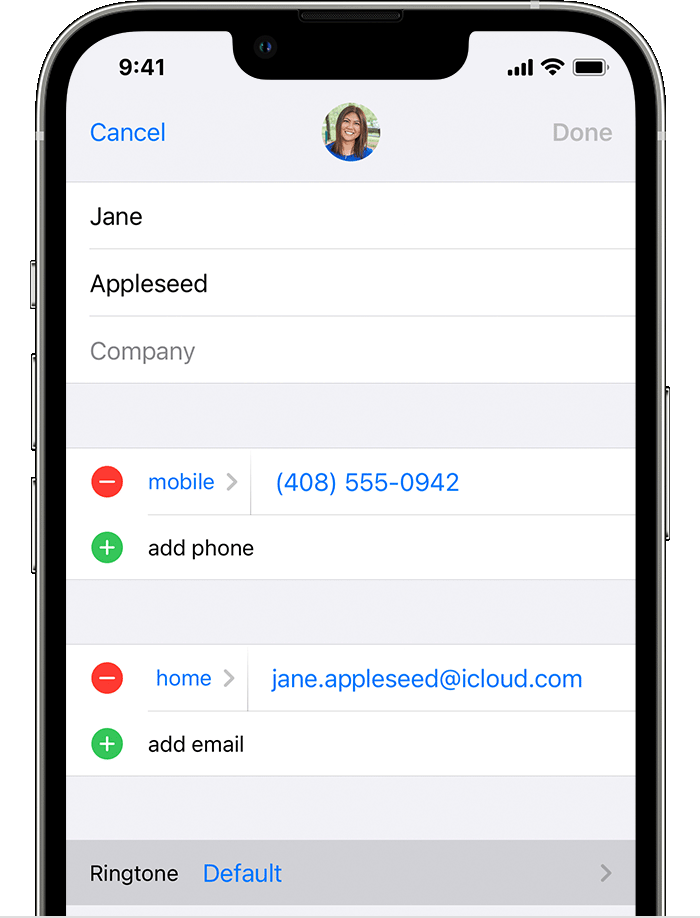The image presented is a high-resolution, portrait-format, color photograph that appears to be a hybrid between a professionally taken photo and a digital animation. This sophisticated, computer-generated graphic showcases the front interface of a sleek, modern smartphone, designed to captivate potential buyers with its sharp and polished look—it exudes a marketing quality.

The smartphone display is shown containing a detailed user profile example. At the top of the screen, the time is marked as 9:41. The profile features a small, circular photo of a young woman with dark skin, possibly of Indian descent, situated centrally. Flanking the photo are two interactive options: "Cancel" to the left and "Done" to the right.

Below the photo, the profile details begin with the first name listed as "Jane" and the last name as "Appleseed." The "Company" field is visible but remains unfilled. Following these are various contact details, starting with a mobile phone number: 408-555-0942, accompanied by an option to add an additional phone number. For her home contact info, the email is listed as jane.appleseed@icloud.com, with an option to add another email address below. At the bottom of the contact information, the ringtone setting is noted as "default."

This image exemplifies the typical settings interface seen within a state-of-the-art smartphone, offering a comprehensive glimpse into how users can personalize their contact details on the device.